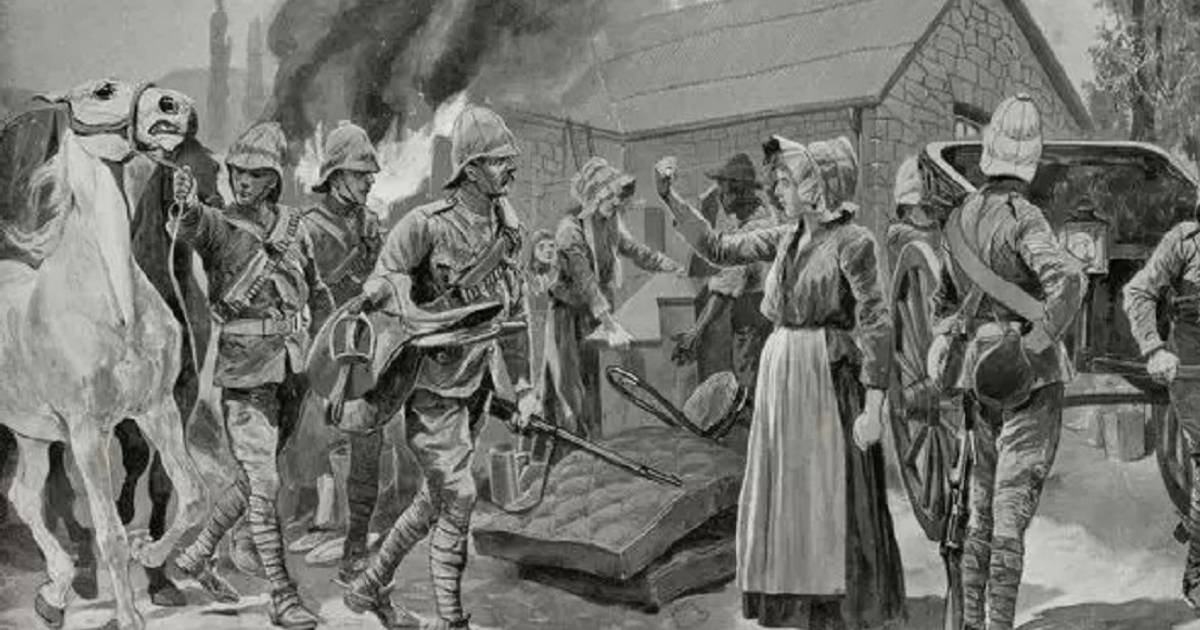In this black-and-white drawing depicting a historical event, we observe a dramatic scene centered around a stone house engulfed in flames on its left side, with thick smoke billowing upwards. The house, flanked by trees, serves as a chaotic backdrop to a confrontation between colonial British soldiers and the home's residents. In the foreground, a soldier pulls a horse buggy while another soldier stands near him, both appearing in heated argument with a woman clad in a bonnet, dress, and apron, who defiantly raises her fist. Scattered around are mattresses, a part of a table, and chairs, suggesting the soldiers are ransacking the house, possibly collecting taxes or evicting the inhabitants. To the left, another soldier stands next to a visibly frightened horse. This vivid portrayal offers a poignant glimpse into the tumult and strife of past conflicts.